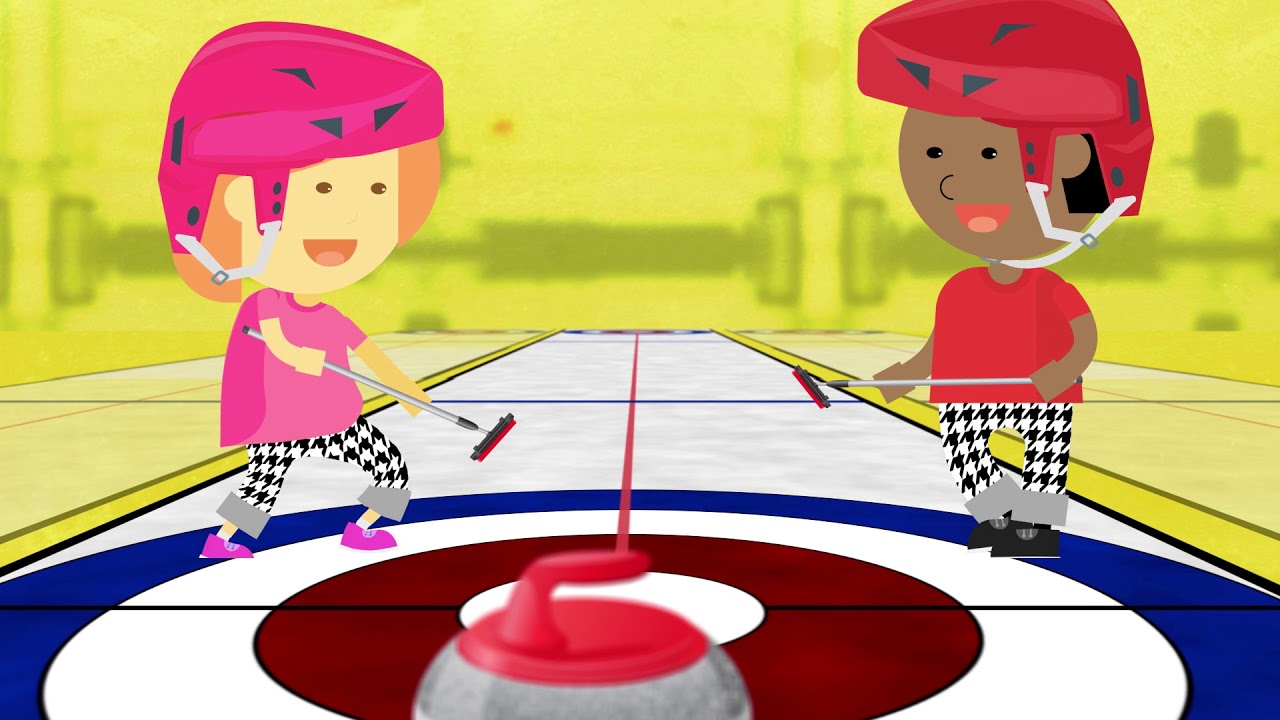This vibrant cartoon portrays two young kids engaging in a game of curling, a winter sport played on ice. The characters, depicted as a girl and a boy, are smiling and energetically wielding their curling brooms. The girl, positioned on the left, has a yellowish complexion, black hair, and is adorned in a pink helmet, pink shirt, and black-and-white cross-hatched pants with gray cuffs. She complements her ensemble with pink shoes. On the right, the boy sports a brown complexion and black hair, matched with a red helmet and a red shirt. He also wears the same patterned pants and black shoes. Both characters are caricatures and are holding cleaning brush-like brooms used in the sport. Central to the scene is the curling stone, a large flat gray disc with a red handle. The ice rink features a bullseye target marked with concentric circles of blue, white, and red, and a prominent red line extends into the background fading towards the vanishing point. The backdrop of the image is primarily yellow, highlighting the playfulness of the scene and the clear focus on the game and the players.